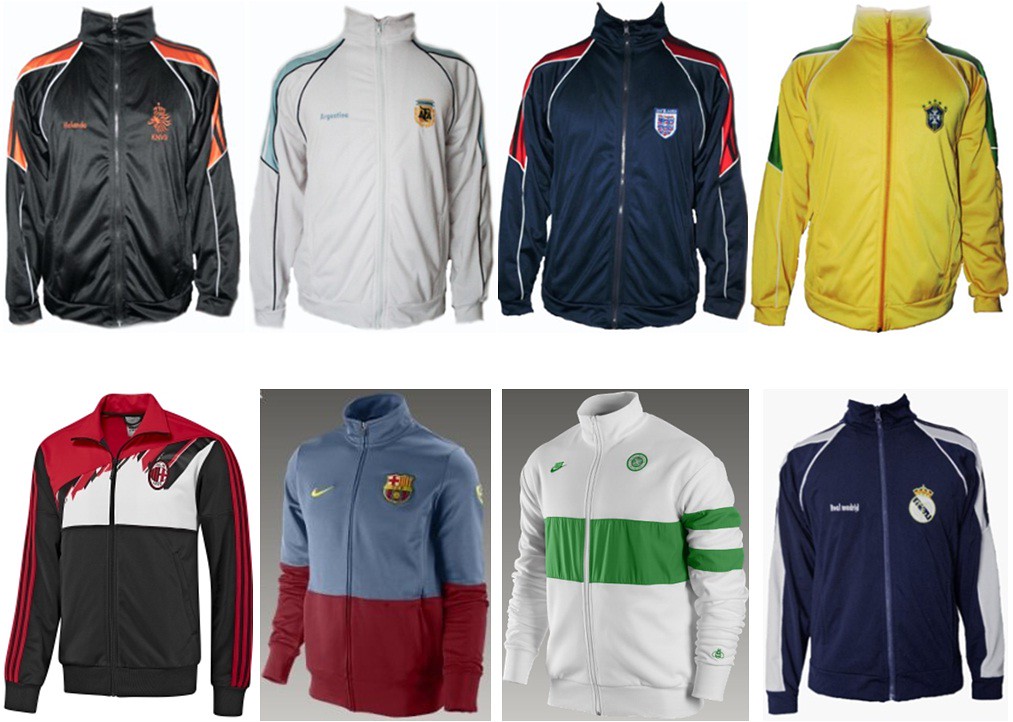The image displays a collection of eight team jackets arranged in two rows of four. Each jacket is a zip-up, long-sleeve design with a collar that can either stand up when fully zipped or fold down when partially zipped. Every jacket features an emblem on the left chest.

**Top Row:**
1. The first jacket on the upper left is black with orange accents on the shoulders and forearms, and it has an orange zipper.
2. The second jacket from the left is primarily white with blue accents on the shoulders and forearms.
3. The third jacket is navy blue with red accents on the shoulders and forearms, and it includes white detailing.
4. The fourth jacket on the far right is yellow with dark green on the shoulders and forearms, and it has an orange zipper.

**Bottom Row:**
1. The first jacket on the lower left is divided into three colors: black on the bottom, white on the chest, and red around the collar. The sleeves are black with red stripes.
2. The second jacket from the left has a maroon lower section and a medium blue upper section and collar. It features a Nike logo on the right chest and an emblem on the left chest, with blue sleeves tapering into maroon at the wrists.
3. The third jacket is predominantly white, with a broad green band across the chest and two green stripes on the left arm separated by a white stripe.
4. The fourth jacket on the lower right is navy blue with white shoulders and sleeves, featuring white stripes running down the arms.

This detailed, photo-quality image appears to be taken from a catalog or a website, showcasing these jackets for potential buyers.